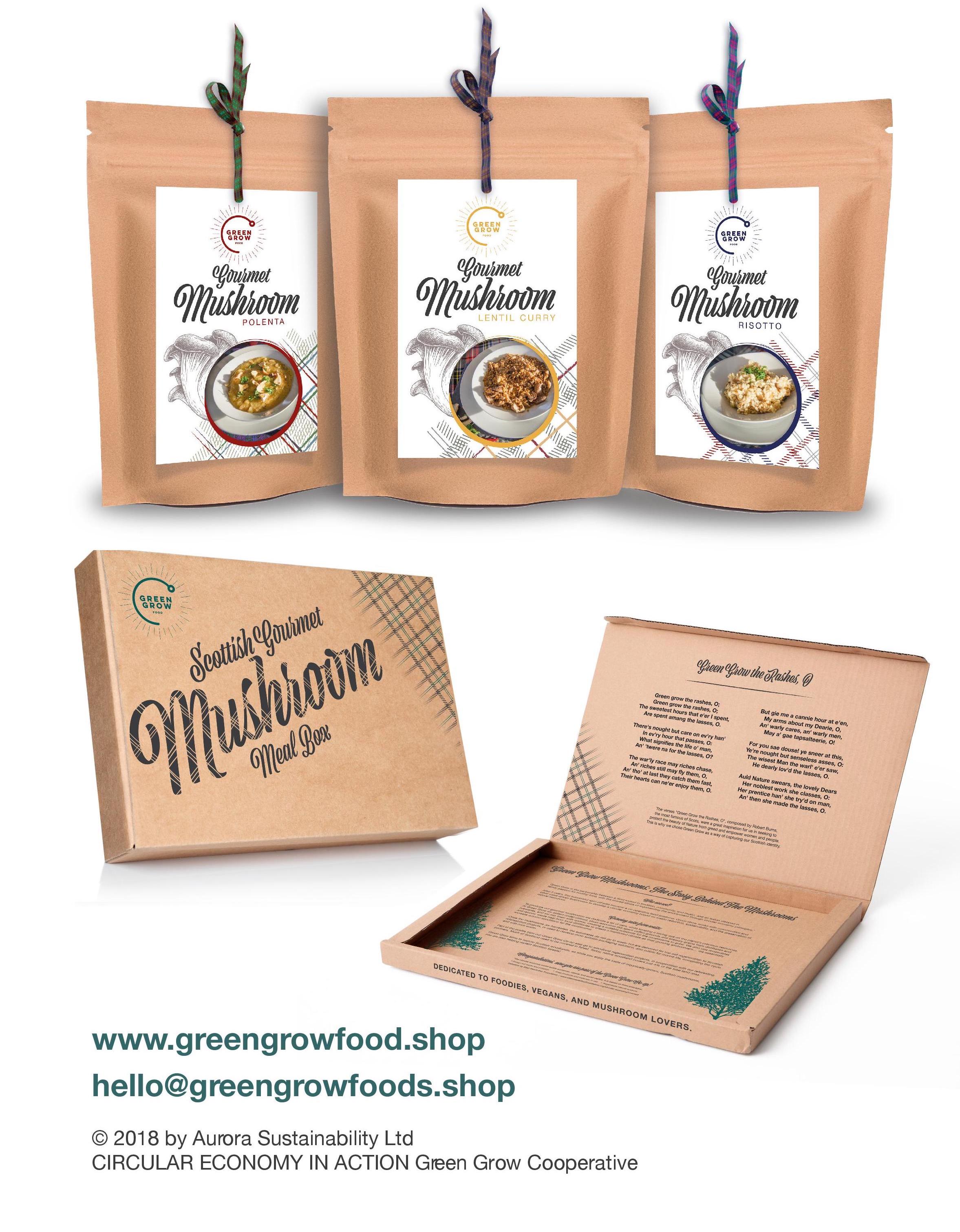The image depicts a product scene of the "Scottish Gourmet Mushroom Meal Box" by Aurora Sustainability, LTD, available through www.greengrovefood.shop. At the top of the image, three tan, cardboard-like pouches are lined up, each with a string attached at the top. The pouches are labeled "Gourmet Mushroom" and feature colorful symbols in red, yellow, and blue, denoting different flavors: Polenta, Lentil Gravy, and Risotto, respectively. Each pouch also showcases a picture of a bowl of food. Below these pouches, there is a brown box, closed and upright on its left edge, which also bears the label "Scottish Gourmet Mushroom Meal Box." To its right, an open box reveals detailed black text on the inside. Additional information is provided on the bottom left corner of the image: "www.greengrovefood.shop" in green text, accompanied by further lines of information about the Green Grove Cooperative and Aurora Sustainability's circular economy initiatives.